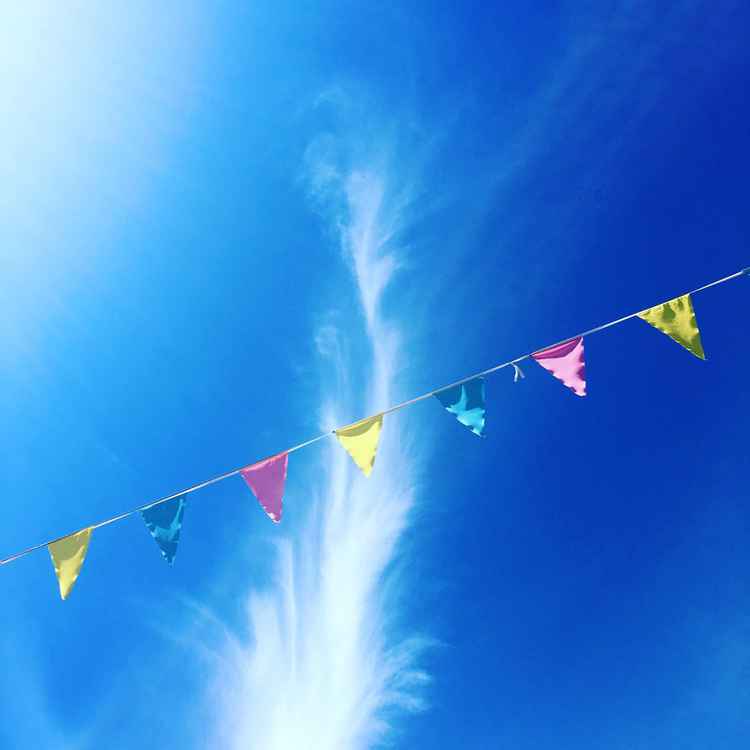In the image, you are looking straight up at a stunning sky that transitions from a vibrant cerulean blue on the right to a lighter blue and aqua hue on the left. The sky features a long, fluffy white cloud in the center, resembling a flame with a thinner middle portion and thicker ends. Hanging across the sky from the left to the right is a string of small, upside-down, triangular pennants. These pennants in vivid hues of yellow, blue, pink, yellow, blue, pink, and yellow add a festive touch, subtly draping from the lower left towards the upper right of the picture. On the right side, the deep ocean-blue sky and a cloud at the bottom create a striking contrast, while the lighter sky on the left displays a hint of white, possibly from sunlight illuminating that area. The scene radiates a serene and celebratory ambiance.